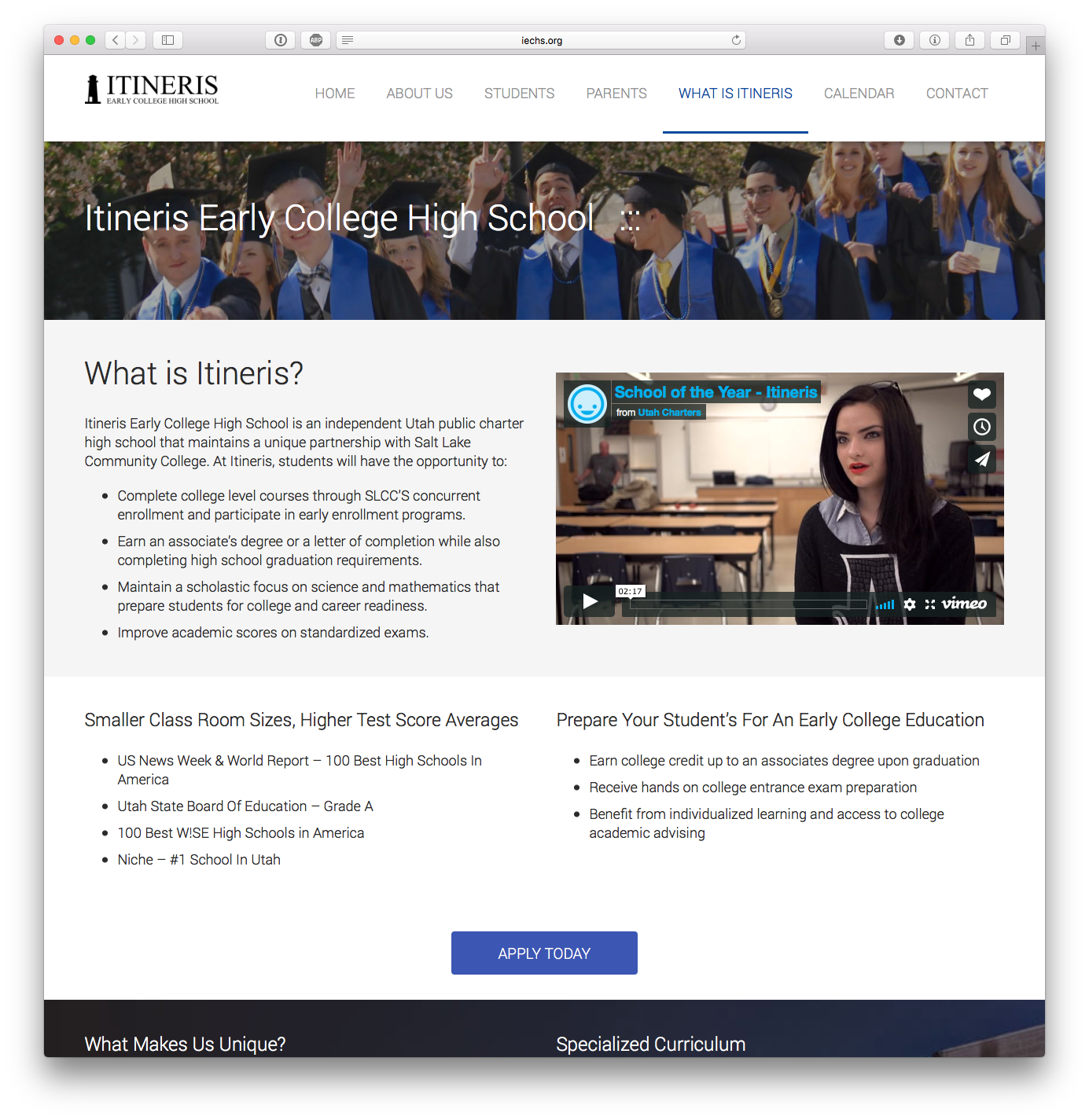This screenshot captures the homepage of the Itineris Early College High School website. In the top left corner, the school's logo is prominently displayed, featuring the name "Itineris" and the tagline "Early College High School." To the left of the logo, an intriguing image resembling a water tower with a cape-like structure flowing to the right adds a unique visual element. 

The user appears to be viewing this site on a Mac, as indicated by the red, yellow, and green window control buttons at the top left of the browser. The web address bar in the middle of the screen displays the URL "IECHS.org," with an information icon situated at the top right for additional page details.

To the right of the logo, a navigation menu lists several tabs: "Home," "About Us," "Students," "Parents," "What is Itinerus" (currently highlighted in blue), "Calendar," and "Contact." The selected tab, "What is Itinerus," opens a section providing information about the school.

Below the navigation bar, the header "Itineris Early College High School" is prominently featured, accompanied by an image of students dressed in black robes, symbolizing their academic achievements and the school's focus on preparing students for college education.